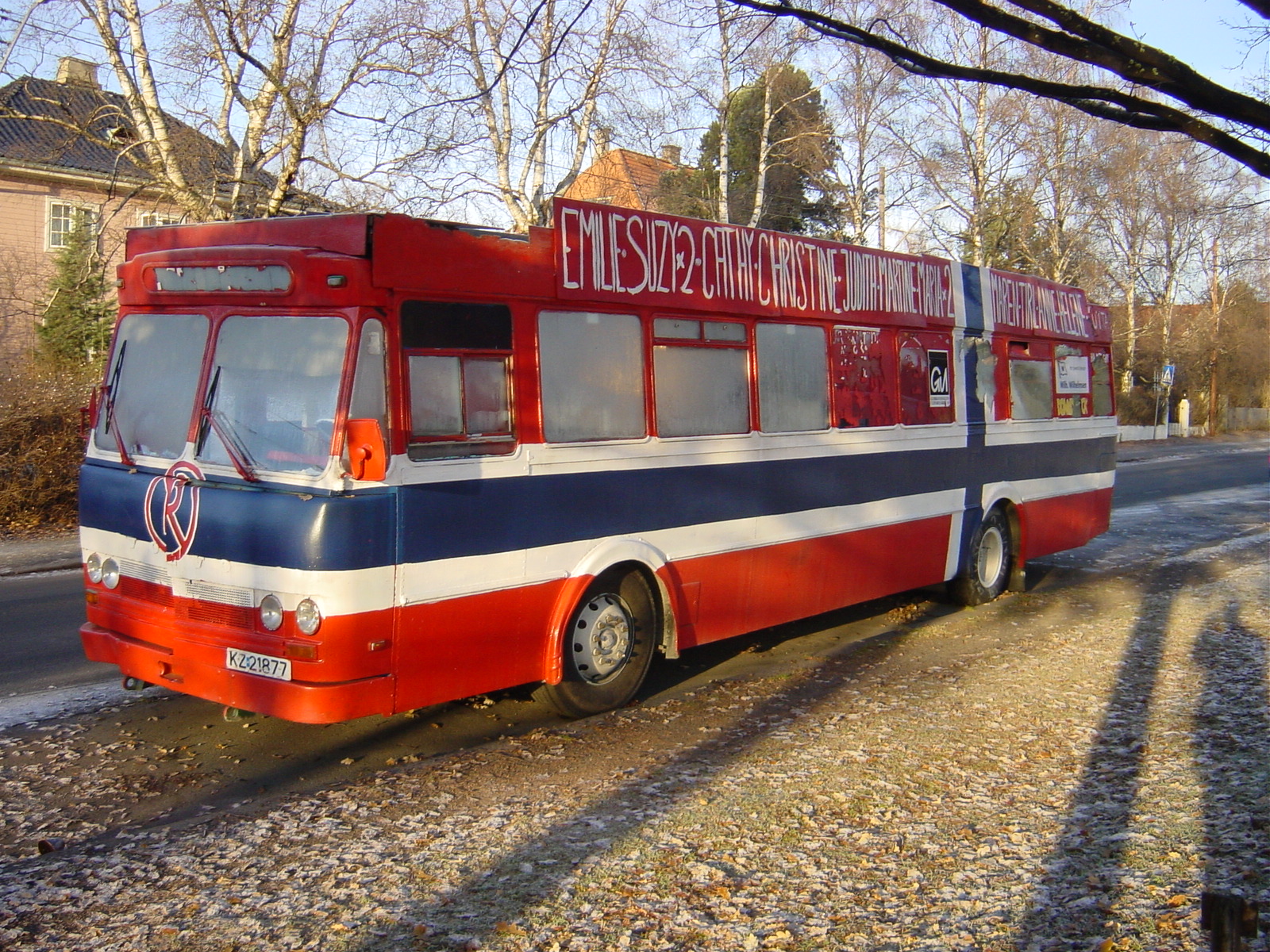A vibrant red, white, and blue bus is parked on an asphalt road in a mostly barren area, where the ground is covered with dirt and scattered dead leaves. The bus features a horizontal color scheme with a red top and bottom, separated by white and blue stripes, and additional vertical stripes near the back wheel. The front of the bus displays a circled letter 'R' in red and a tag below the headlights. White letters and numbers, written in a foreign language, are visible on top of the bus. Its windows are blacked out, and it appears to be a personalized vehicle, possibly repurposed. Surrounding the bus are trees mostly devoid of leaves, suggesting it's winter, with a few pine or cedar trees standing out. Red brick houses with various roof colors—black, brown, and red—are visible on the other side of the road, along with small, unreadable signs.